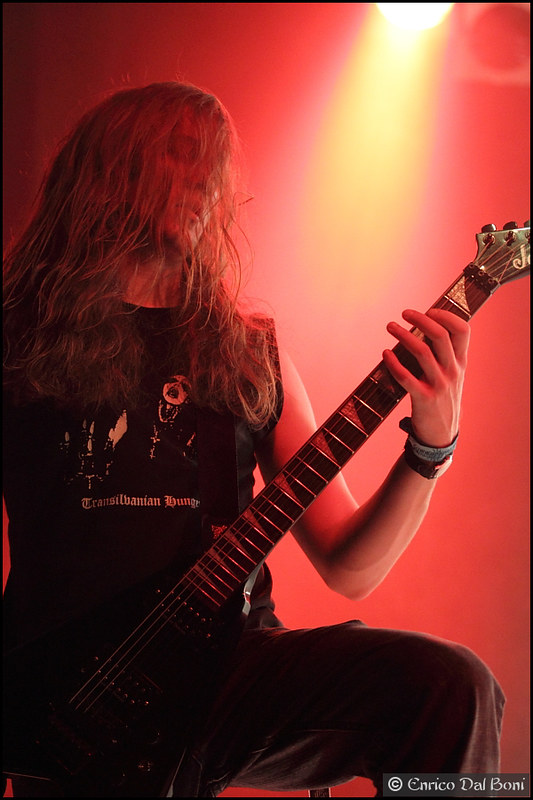A close-up photograph captures a hard rocker, unmistakably Caucasian, deeply engrossed in playing an electric guitar on stage. The performer, with long, wavy hair cascading past his shoulders and partially obscuring his face, exudes an intense, metal-inspired aura. His eyes are shut, reflecting his immersion in the music. Clad in a sleeveless black shirt bearing the text "Transylvanian Lounge" and adorned with a monster graphic, the rocker also wears dark brown pants, a wristwatch, and multiple bracelets. His black vest prominently features a metal logo. He grips the fretboard of his guitar with his left hand and stands near a stool with his left leg bent. The background radiates various shades of red, illuminated by a yellow spotlight above and augmented by the stark white light shining down, casting a dynamic ambiance. The image is imbued with an overall reddish hue, emphasizing the intensity of the moment. The photograph, marked "Copyright Enrico Dalboni" at the bottom, captures the raw energy and emotion of the performance.